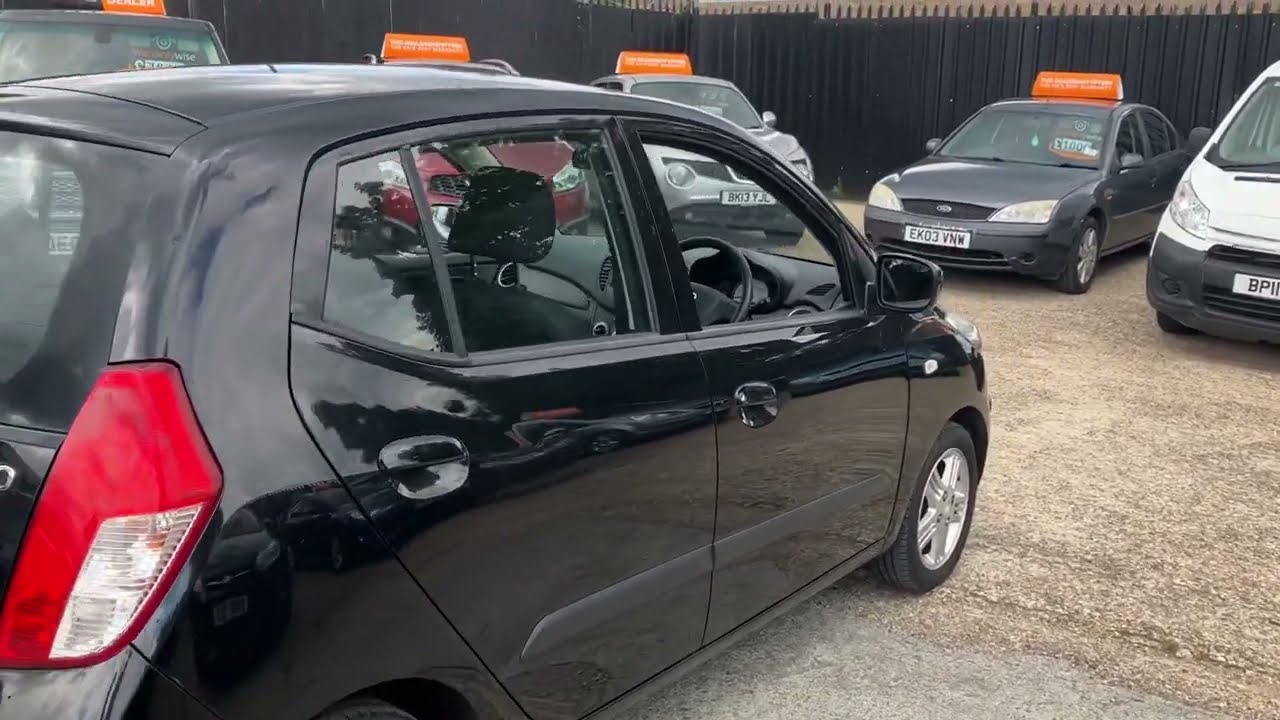The image depicts an outdoor car lot during daytime, primarily occupied by a black four-door hatchback compact car positioned in the foreground, facing away from the viewer. The car is notable for its right-hand drive configuration, as evidenced by the visible steering wheel through the open window on the driver's side. The car is parked on a surface mostly covered in brown gravel, with a slight indication of gray pavement at the bottom of the picture. 

In the lower left, the red and white taillight of the hatchback is visible, and a black fence forms the backdrop behind the row of vehicles. Surrounding this black car are multiple other vehicles facing towards it: some with orange signs on their roofs featuring indiscernible white lettering, suggesting they might be taxis. These vehicles include a mix of different styles and colors: a gray car, a silver car, a maroon red car, a black truck, a white van, and a silver jeep-like vehicle. Each car has a thick white license plate affixed to its front bumper. The overall composition places the black hatchback at the center of attention amid a diverse background of other vehicles.